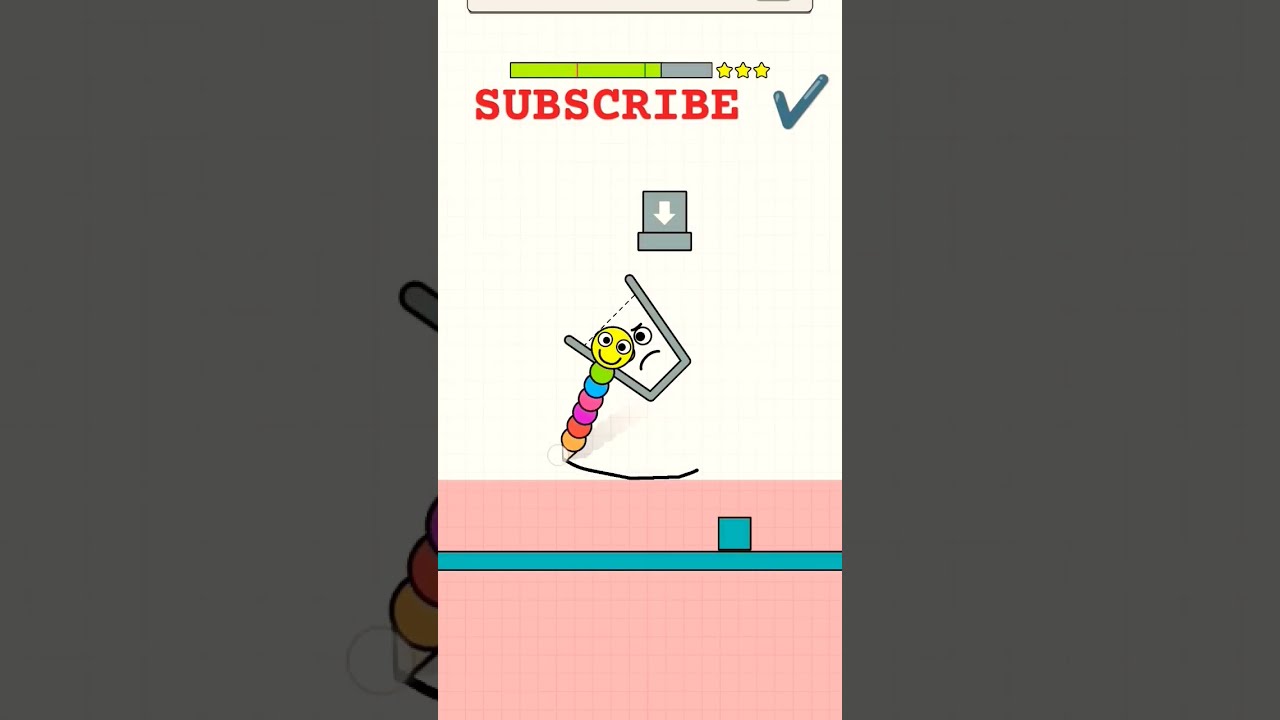The image is a detailed screenshot from a video, possibly from a mobile game, asking viewers to subscribe to a channel. The central portion of the screen is dominated by a white background, giving way to a light pink section at the bottom third. A turquoise stripe runs horizontally across the pink section, incorporating a turquoise square on its right side. In the center, there is a unique caterpillar-like figure, resembling a multicolored pen, with orange, red, purple, pink, blue, green balls in sequence, and a larger yellow circle with a smiley face at the top. This figure is drawing a curved line. Adjacent to it, on the left, is a tipped-over trash can with a frowning face, sharing an eye with the pencil caterpillar character.

At the top sits a rectangular horizontal meter bar, predominantly in green, indicating a health or progress status, with roughly three-quarters filled. Three yellow stars are positioned to the right of the meter bar. Below this, in bold red letters, the word "SUBSCRIBE" is prominently displayed, followed by a blue check mark. Directly beneath the "SUBSCRIBE" text is a grey box with a white arrow pointing downward, likely symbolizing a download or further action prompt. The borders on the left and right thirds of the image are dark, contrasting with the lighter central section.